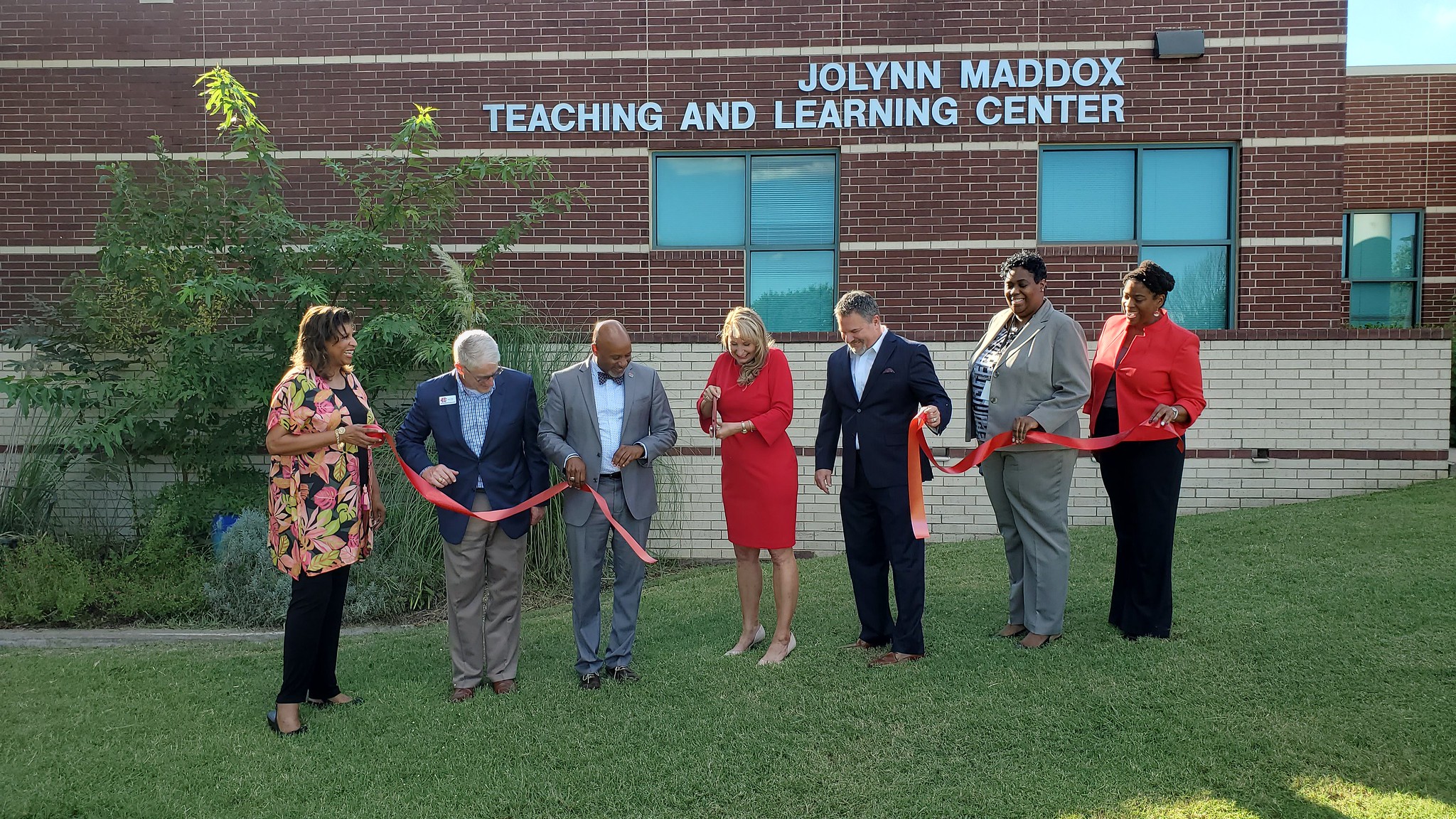The image captures a ribbon-cutting ceremony for the Jolin Maddox Teaching and Learning Center. In the foreground, seven individuals stand side by side on grass, with a plant to the left. Central to the image is a woman in a red dress, holding a large pair of scissors, poised as if she has just cut the red ribbon. Flanking her, on her left, are a woman and two men holding one part of the ribbon, while on her right, a man and two women hold the other part. They are dressed in a variety of suits and dresses in colors such as tan, brown, gray, blue, green, red, pink, and black. Behind them, the building's wall is visible, constructed of white bricks at the bottom and ruddy brown bricks above. The building features several windows, including two shaped like an upside-down L with three window panes each. The white text on the brick wall reads "Jolin Maddox Teaching and Learning Center." The overall setting is outdoor, in the daytime, with light green grass and plants contrasting with the blue sky reflected in the windows.